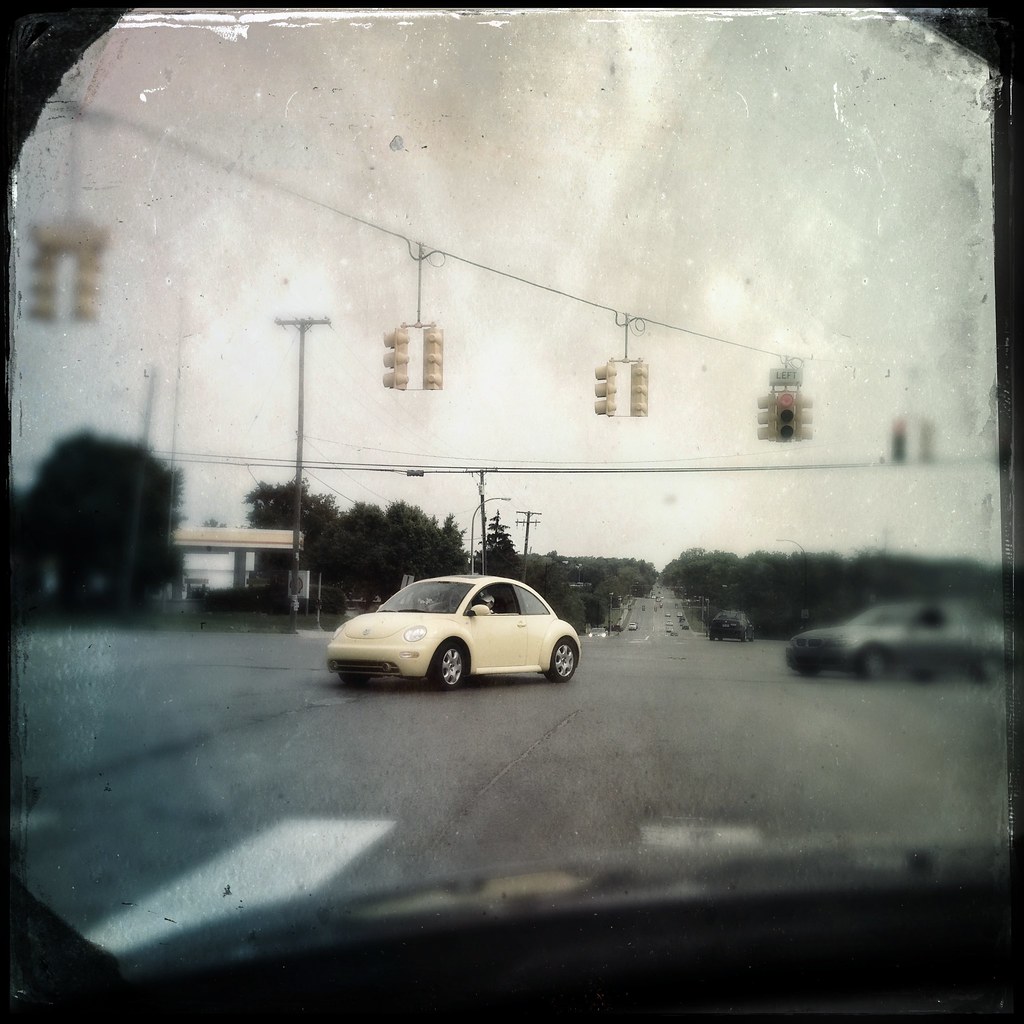The distressed sepia-toned photograph is viewed through the front windshield of a car, with all four corners darkened, giving the image a vintage feel. Central to the scene is a yellow Volkswagen Beetle with its windows open, moving towards the photographer. Directly in front of the Beetle is a crosswalk. To the left, slightly behind the Beetle, stands a gas station, while a dark-colored, potentially silver or gray BMW is positioned to the right, also trailing the Beetle. Overhead, five yellow traffic lights hang from a power line, with two lights facing the camera displaying red signals, and one marked with a "left" turn sign. In the background, additional cars are visible, hinting at approaching and receding traffic on the roadway. The windshield wipers and part of the dashboard frame the photograph, suggesting it was taken from within a vehicle, capturing a mundane yet intriguing streetscape.